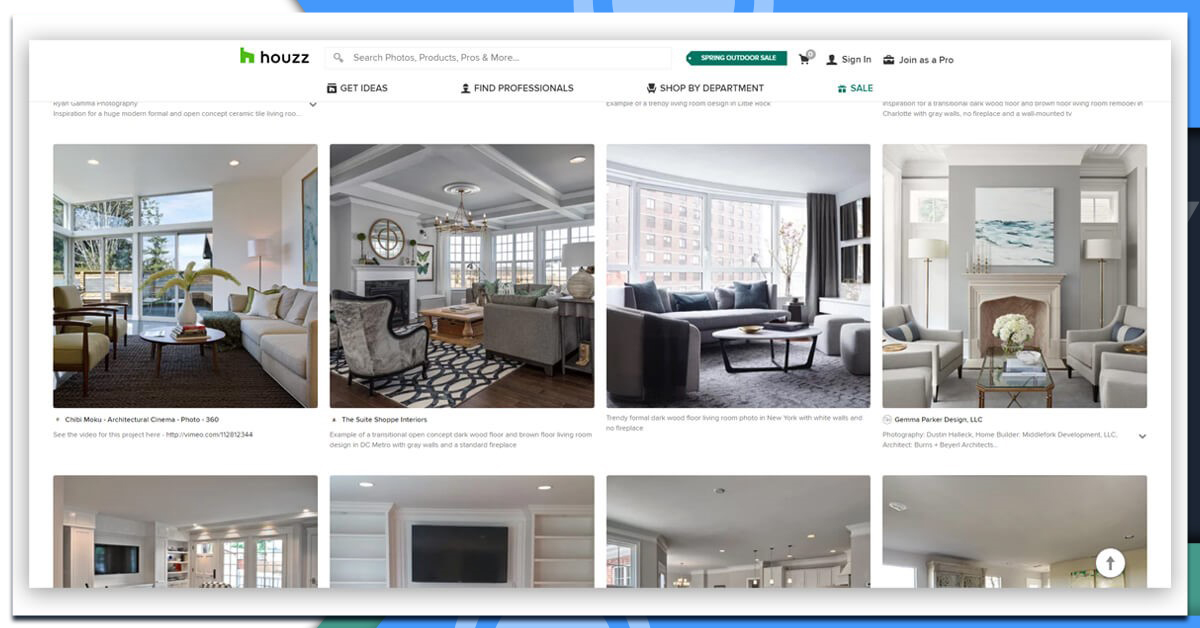This image is a website homepage for Houzz, displayed on a computer screen. Houzz, spelled H-O-U-Z-Z, is identified by its green 'H' symbol positioned in the middle toward the left corner. The website focuses on interior decorating and real estate, showcasing a variety of photographs depicting interiors of houses and apartments. Users can see options to shop sales, sign in, or join as a pro. Navigation tabs include sections such as "Get Ideas," "Find Professionals," "Shop by Department," with a prominent banner advertising a sale, illuminated in blue. The interface predominantly highlights modern furniture presented in diverse color palettes.

The website design features a blue bar spanning three-quarters of the top part of the page. This bar curves downward, transitioning into a brown bar, following the curvature down to the bottom. Although the blue bar dominates, interruptions in the imagery occur: notably, four of the displayed pictures are only partially visible, as they're cut off at the bottom. Overall, the website blends visual elements of both functionality and aesthetics, emphasizing modern interior design.